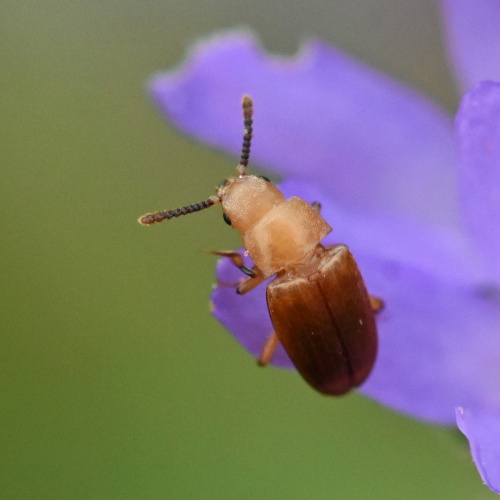This detailed close-up photograph showcases a brown beetle with a darker brown covering on its back and a lighter honey brown body. The beetle's head features two black eyes and antennas extending to the sides. Its legs, six in total, grip the edge of a vivid purple flower. The beetle appears magnified in the photograph, highlighting every intricate detail of its body, head, and legs. The background is an abstract blur of green, ensuring the beetle and the purple flower are the focal points of the image, providing a sharp contrast to the soft, out-of-focus backdrop. Notably, the beetle has a dark line running down its middle, possibly where its wings open up, and its legs appear slightly darker at the edges. The photograph captures the beetle positioned diagonally, from the upper left to the lower right.